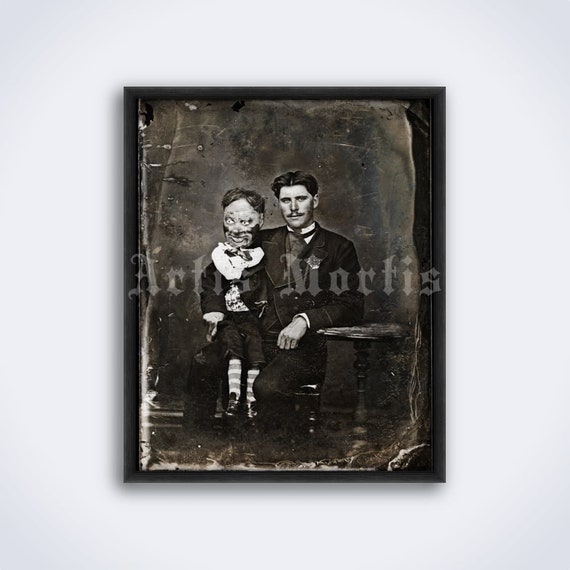This is a detailed black-and-white photograph, itself a meticulously crafted reproduction that evokes the look of an aged and torn vintage image. The photograph is encased in a black frame and mounted on a plain white wall. Centered in the composition, a man with fair skin and dark hair, parted neatly down the middle and slicked back, gazes directly at the viewer. He sports a thin black mustache and dark eyebrows, complementing his old-fashioned black suit adorned with a high white collar and a cravat-like tie. 

Seated in a wooden chair, his left arm rests on a round wooden table beside him, while his right arm supports a ventriloquist's dummy perched on his right thigh. This dummy bears a striking resemblance to its handler, with exaggerated facial features including facial hair that mimics the man's mustache and ragged clothing that mirrors the man's suit. The dummy's attire includes a dark suit, short pants, striped socks, and black shoes, lending it an eerie, lifelike appearance. The expression on its face is unsettling, and it seems to have some unnatural substance smeared across its features. 

The entire scene is positioned against a plain background, further emphasizing its surreal and haunting quality. Overlaying the photograph, in a light, almost spectral script, are the words "Artis Mortis."